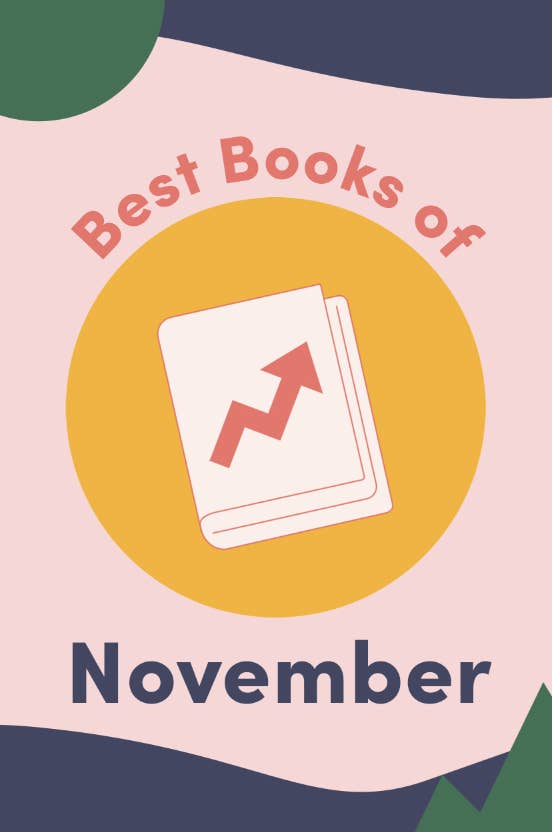The image is a vibrant, graphic art-style poster promoting "The Best Books of November." At the center of the poster is an orange circle featuring a white book with a pink arrow pointing upwards, symbolizing an increase in book sales. Encircling the central image, the phrase "Best Books of" appears above the circle in pink, with "November" below in a deep, matching purple.

The background is a vivid pink, embellished with various geometric shapes including green circles and triangles. The upper left section of the background showcases a light green circle, while the top right corner and areas around the lower part of the poster are filled with deep purple. Additionally, the bottom right corner of the poster includes two green triangles that resemble mountains, aligning with the green circular design at the top left. The top and bottom borders are also accented in deep purple, creating a cohesive and eye-catching design.